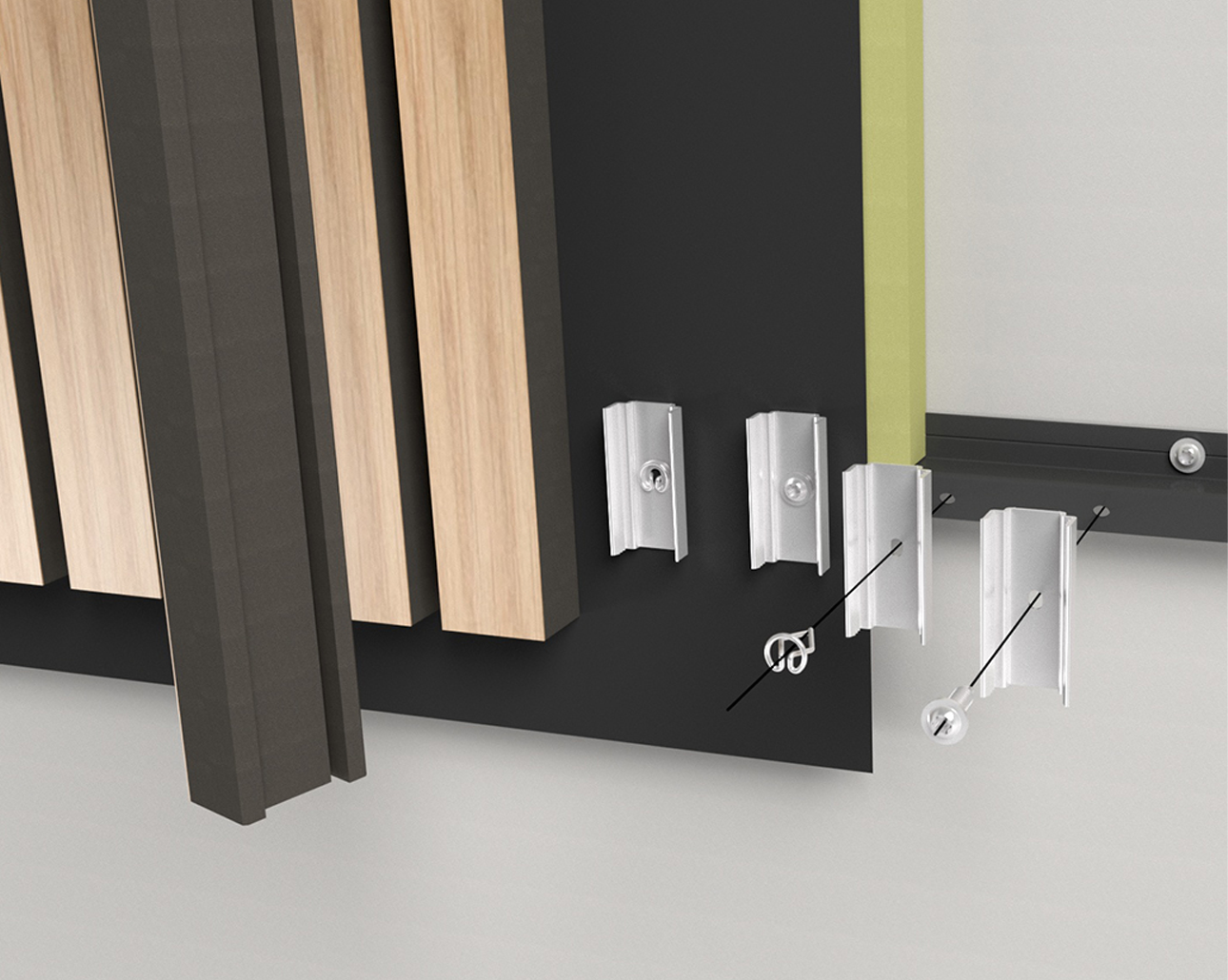This photograph showcases a detailed close-up of a wall-mounted paneling system, likely part of a showroom or design studio display. Central to the image is a section of light gray linoleum-style flooring, bordered by the black track system at the base of a white wall. The wall features several vertical wooden slats in both light and dark finishes, highlighting various paneling options. Adjacent to these slats is a lime green vertical post, supported by aluminum brackets designed for mounting. These brackets, silver in color, provide a glimpse into the installation process, showing inserts that affix into the floorboard against the wall. Also visible is a slightly extended gray pillar that resembles an I-beam, possibly part of the structural display. The entire setting is enclosed within what looks like a square frame, forming a neat and organized presentation. The background, a dark chocolate brown with a green trim, contrasts the lighter paneling options, adding depth to the display. Additional instructional elements such as directional arrows and mounting hardware tips are shown, presumably to demonstrate the assembly and installation method. It’s an informative setup, ideal for educating viewers on the construction and aesthetic possibilities of this wall paneling system.